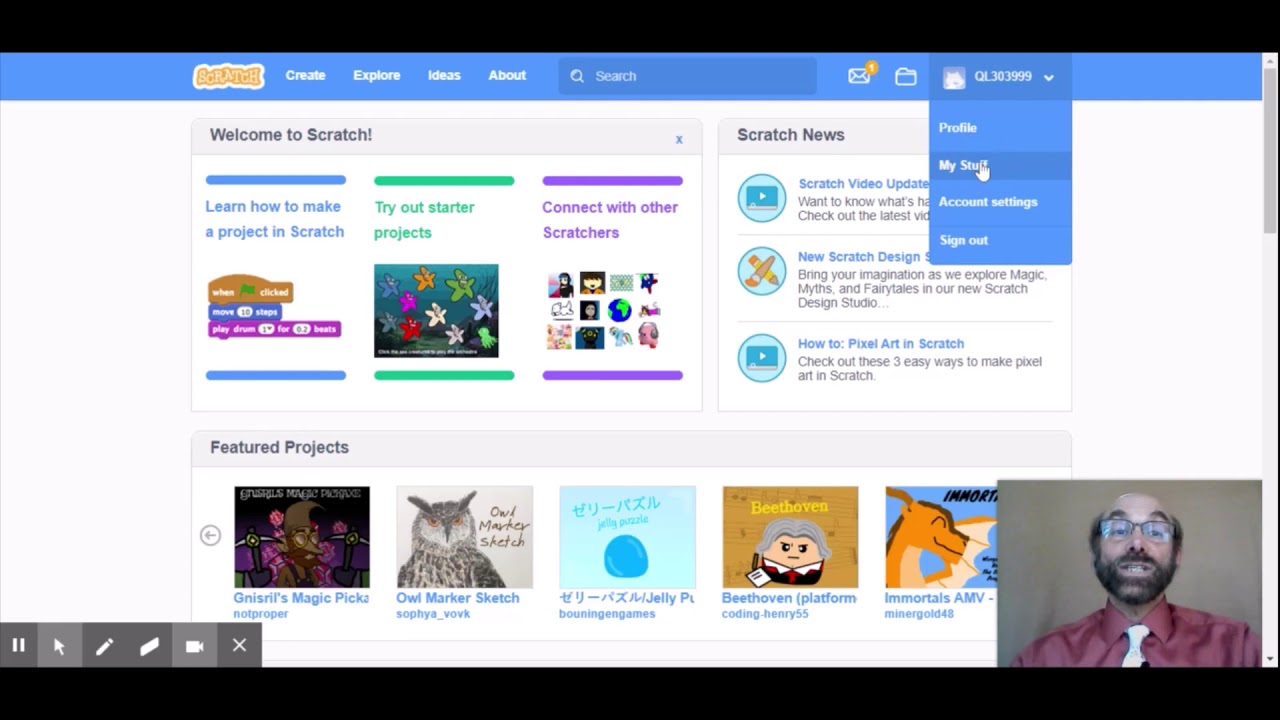The image depicts an online class interface with various interactive elements and sections. In the bottom right corner, there is a picture of an instructor or tutor, wearing a purple t-shirt and a white tie, indicative of a live class session. Below the tutor's image, at the bottom left, several control buttons are visible: Pause, Cursor, Pen, Eraser, Read, Document, and Close. The interface's background is blue.

In the top left corner of the interface, the heading says "Scratch" in orange. Additionally, there are several tabs such as "Create," "Explore Ideas," "About," along with a search bar, mail icon, folder icon, and a user profile icon. The user profile icon has been clicked, revealing a dropdown menu with the options: Profile, My Stuff, Account Settings, and Sign Out.

The layout of the page is divided into three main sections:
1. **Welcome to Scratch**: This section includes links such as "Learn how to make a project in Scratch" (in blue text), "Try out starter projects" (in green text), and "Connect with other Scratchers" (in purple text).
2. **Scratch News**: This section contains updates and news related to Scratch, with various titles:
   - "Scratch Video Update" (partially obscured by the profile icon)
   - "New Scratch Design: Bring your imagination and explore magic, myth, and fairy tales in our new Scratch Design Studio"
   - "How to Pixel Art in Scratch: Check out these three easy ways to make pixel art in Scratch"
3. **Featured Project**: This section showcases a project titled "Genie's Trails," with additional tags such as Magic, Picard, Nandrofa, Sketch, Burning, Games, and creators including Bet, Hoven, Coding, Henry55, Immortal MV, and Bimanagold48.

Overall, the image provides a comprehensive overview of an educational platform, highlighting an online class, user interaction tools, Scratch-related news, and featured projects.